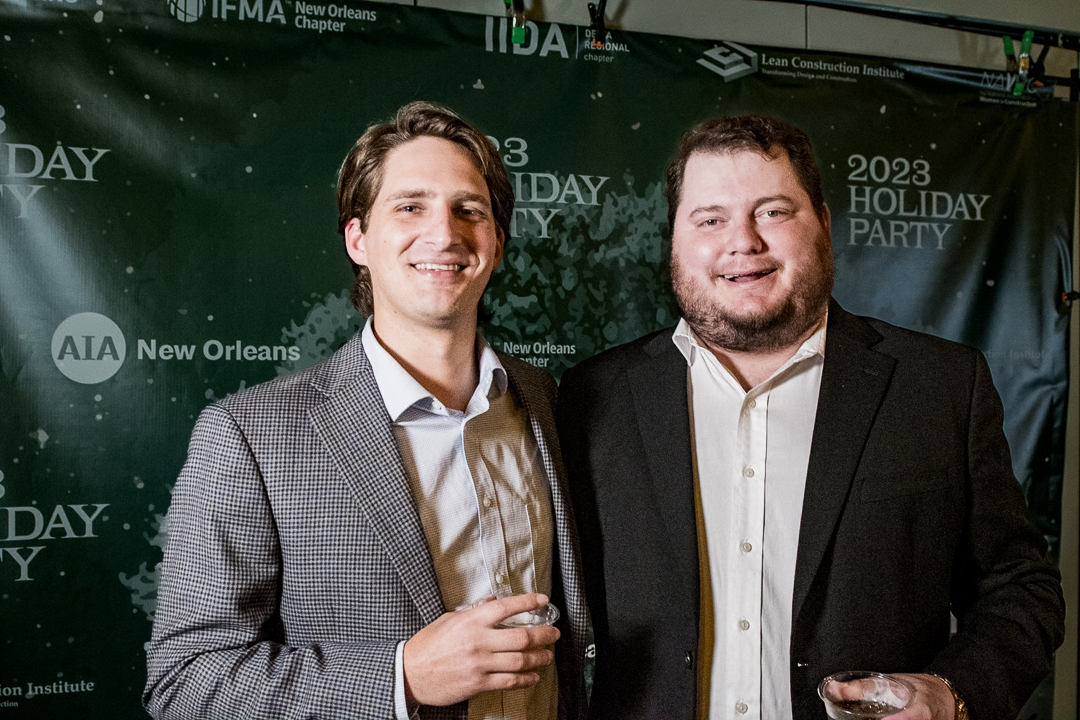In this photograph, two men are standing side-by-side, posing together at what appears to be a festive event. The man on the left, a white male with brown hair, is smiling at the camera. He is dressed in a white button-down collared shirt under a gray wool blazer, holding a plastic cup in his hand. The man next to him, also white, has dark black hair and a scruffy beard. He too is dressed in a white button-down collared shirt, paired with a black blazer, and is holding a plastic cup while smiling at the camera. Behind them is a prominent wall with a green banner that reads "2023 Holiday Party AIA New Orleans," adorned with various graphics in shades of black, white, and gray.